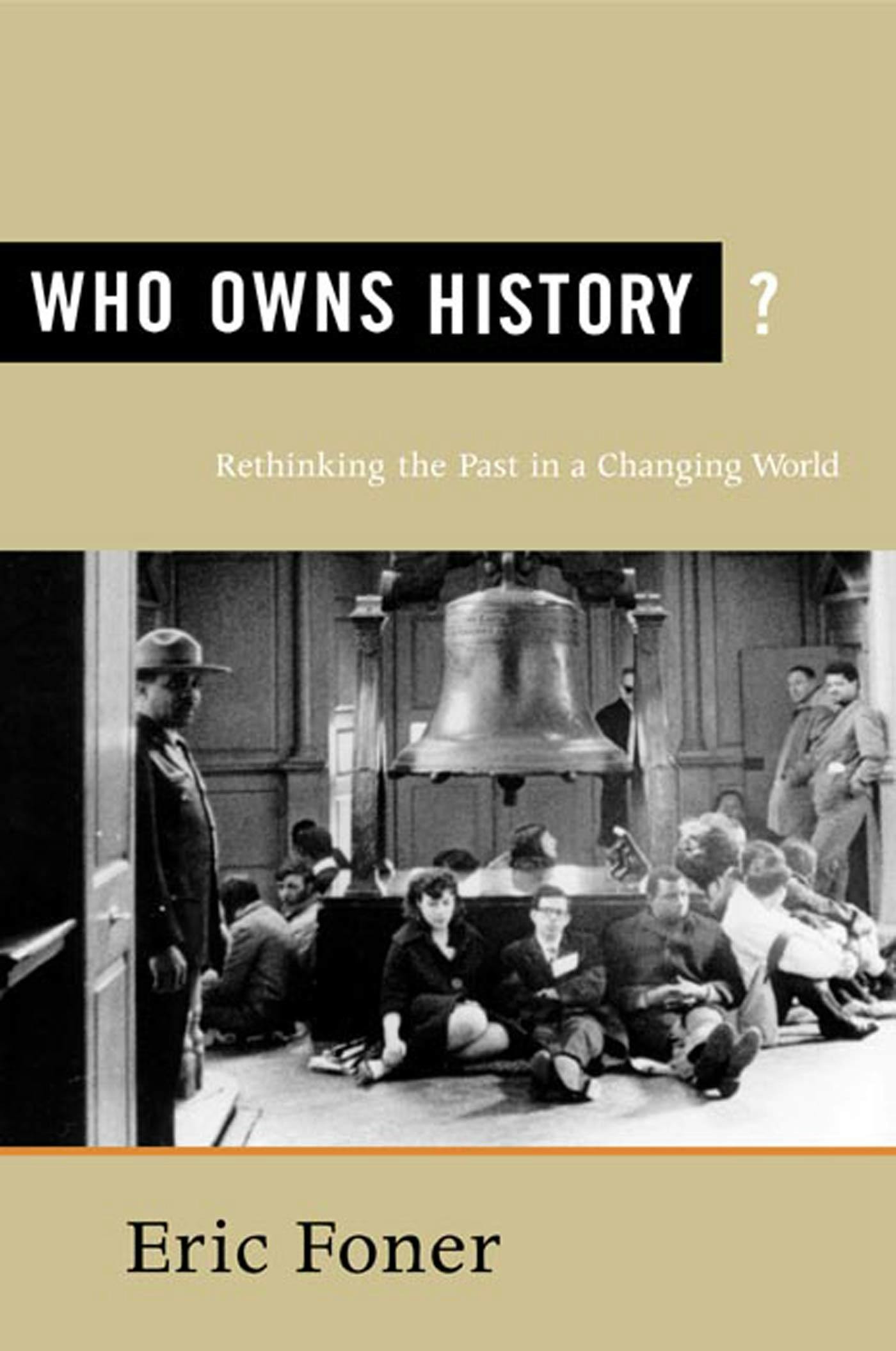The image is a detailed cover of a book, characterized by its vintage, retro aesthetic. The background is a tan color, adding to its old-fashioned appearance. Dominating the top of the cover is a black rectangle, within which the title "Who Owns History?" is inscribed in white font, with a distinct question mark placed just outside the black banner. Beneath the title, also in white font, is the subtitle "Rethinking the Past in a Changing World."

Central to the cover is a striking black and white photograph, likely from the 1960s, depicting a sit-in protest at the iconic Liberty Bell. The image features various individuals, including people seated around the bell, two individuals standing in the corner, and another person in the doorway. Adding context to the scene, there are viewers including workers and possibly a park ranger, identifiable by their attire, such as jumpsuits.

An orange line stretches across the bottom part of the cover, separating the photograph from the author's name, "Eric Foner," which is displayed below in black text. The combined elements of typography and imagery convey a thoughtful reflection on historical narratives in contemporary society.